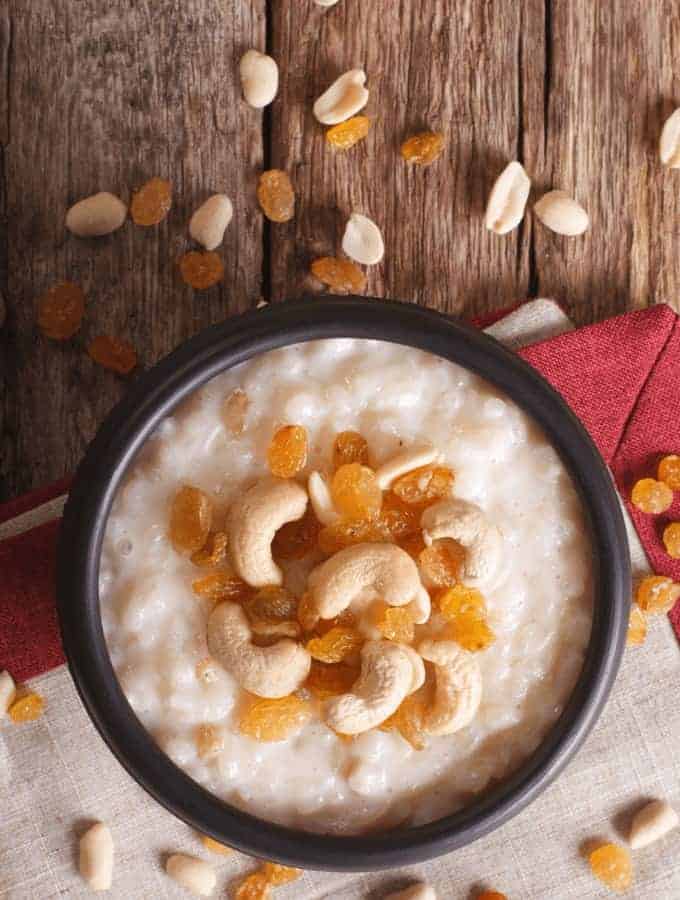The image features an overhead view of a black bowl filled with a white creamy porridge or pudding. The porridge is generously topped with light brown, crescent-shaped nuts, likely cashews, and yellowish, raisin-like dried fruits. These toppings also appear scattered around the bowl on a red and white placemat. The placemat itself is set on a surface of brown wooden planks. In the surrounding area on the table, more loose nuts and dried fruits are dispersed, adding to the rustic and appetizing presentation.